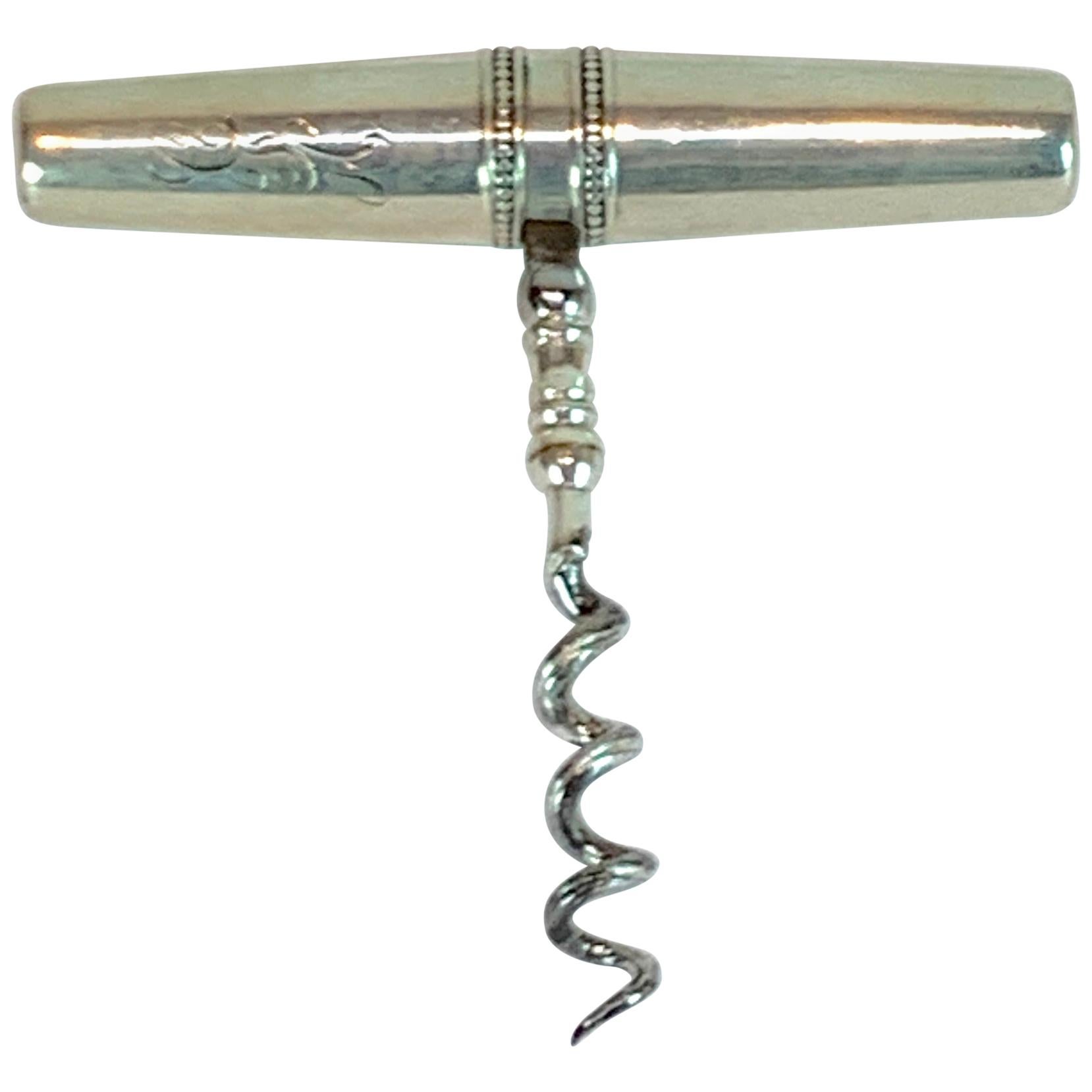This image features a vintage, ornately crafted corkscrew made entirely of polished silver. The corkscrew stands approximately three inches tall and boasts an elegantly long handle designed for a firm grip. The handle is adorned with intricate carvings on one side, and features two bands embellished with small dots or possibly rhinestones, running around its circumference near where the screw begins. Between these bands and the screw are globe-like or orb-shaped structures that add to its ornate appearance. The actual screw itself has precisely four spirals, ending in a sharply pointed tip ideal for piercing and extracting a wine bottle cork. The entire corkscrew is highly reflective and displayed against a white background, further highlighting its sleek and shiny silver finish.